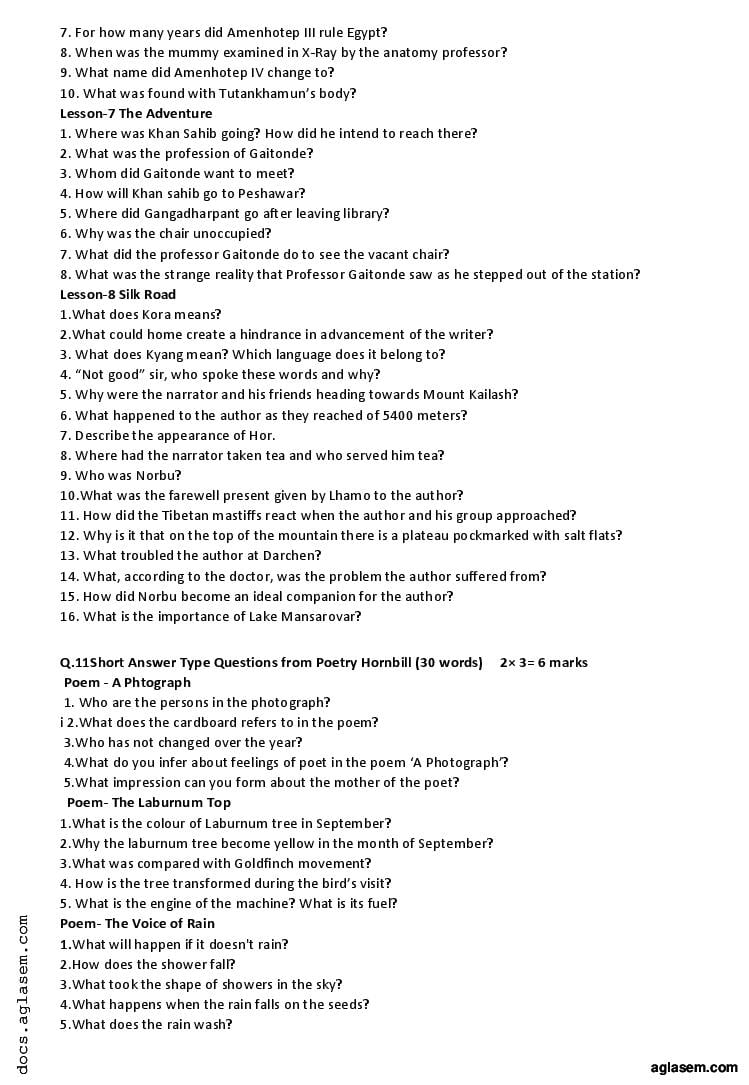In the image, multiple questions are presented, presumably related to a lesson or passage from "Silk Road, Lesson 8". The questions include:

1. What was the profession of Gaitandi?
2. Whom did Gaitandi want to meet?
3. How will Khan Sahib go to Peshawar?
4. Where did Gangadhar Pant go after leaving the library? Why was the chair unoccupied, and what did Professor Gaitandi do to the vacant chair?
5. What strange reality did Professor Gaitandi encounter as he stepped out of the station?
6. What is the meaning of "Quora" and how might it create an obstacle in the writer's progress?
7. What is the meaning of "Qiang" and which language does it belong to?
8. Who said "Not good sir" and why?
9. Why were the narrator and his friends heading towards Mount Kailash?
10. What happened to the author at 5400 meters and describe their appearance of horror?
11. Where had the narrator taken tea and who served it?

These questions cover various aspects like characters, their actions, the meanings of words, and specific events that appear to be pivotal within the lesson they are extracted from.